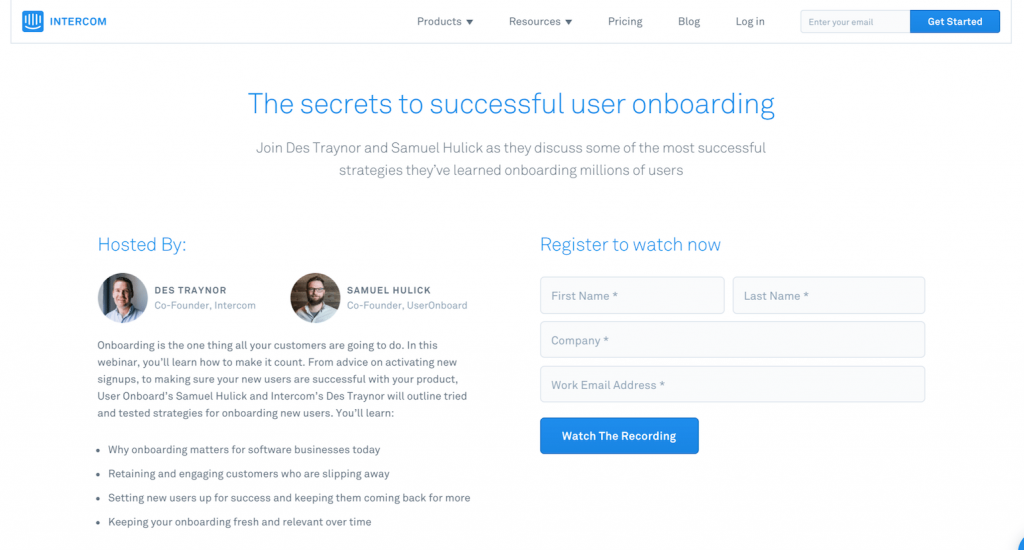**Descriptive Caption:**

The image is a detailed section from the Intercom website. In the top left corner, there's a small blue square with rounded edges featuring five vertical lines above a curved line resembling a smiley face, next to the word "INTERCOM" in all caps. On the far right of the header, there are grey drop-down menus labeled "Products" and "Resources," followed by links to "Pricing," "Blog," and "Login." Further along, there's a field for entering an email address accompanied by a blue "Get Started" button.

The main screen has a white background with a prominent blue header reading "The secrets to successful user onboarding." Below it, in smaller grey text, it says, "Join Dez Trainer and Samuel Hulik as they discuss some of the most successful strategies they've learned onboarding millions of users." 

Directly underneath this text, there are small profile pictures of Dez Trainer, co-founder of Intercom, and Samuel Hulik, co-founder of User Onboard, under the heading "Hosted by." 

Following this, the presentation explains: "Onboarding is the one thing all your customers are going to do. In this webinar, you'll learn how to make it count, from advice on activating new signups to ensuring your new users are successful with your product." It details further topics covered in the webinar: 
- Why onboarding matters for software businesses today
- Retaining and engaging customers who are slipping away
- Setting new users up for success and keeping them coming back for more
- Keeping your onboarding fresh and relevant over time

Finally, there's a prompt to register to watch the recording. It requires entering a first name, last name, company, and work email address, and concludes with a blue "Watch the Recording" button.